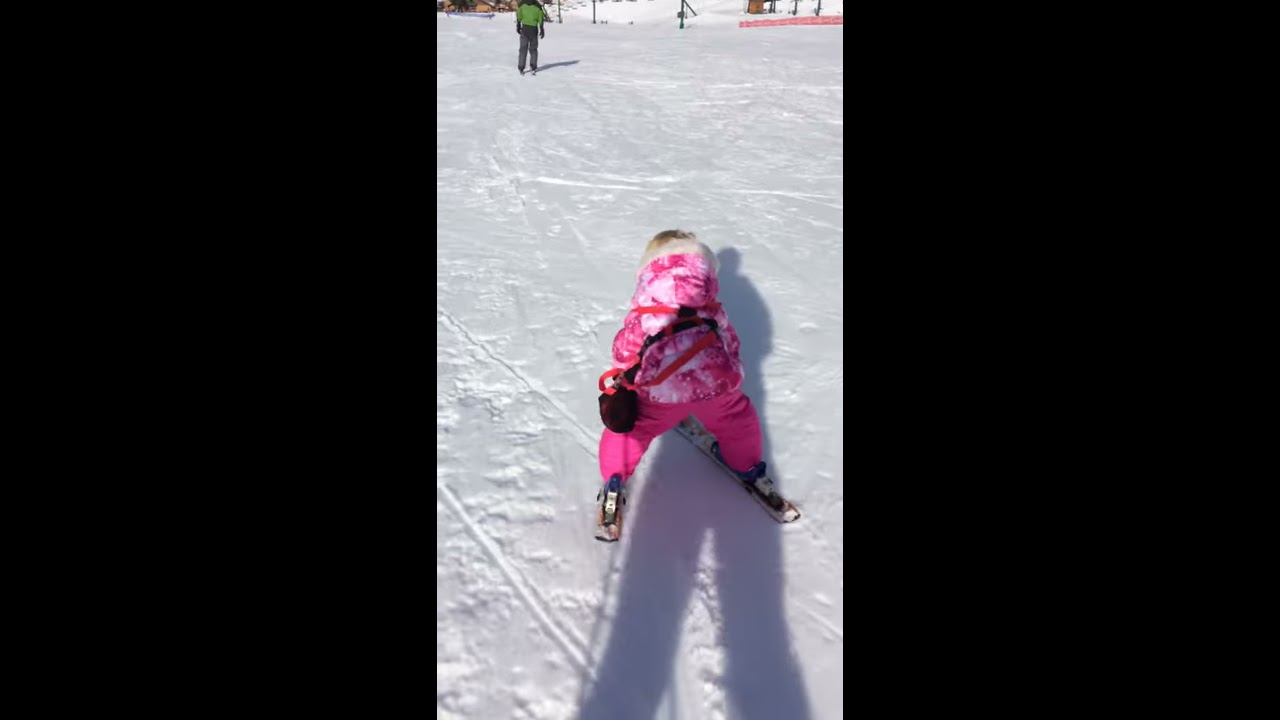This detailed photograph is presented in a triptych style, with the left and right panels featuring solid black backgrounds. The central panel captures a snowy scene at what appears to be a ski resort. The focal point of the image is a small child, likely a toddler, seen from behind. She has blonde hair and is wearing pink pants along with a pink and white jacket. The child is equipped with skis and appears to be attempting to walk or ski, facing slightly to the right. Her attire includes a white and pink hat and a pink face covering, complemented by black gloves on her hands. The child carries a small bag on her back.

Distinct shadows, presumably cast by the person taking the photograph, stretch across both the child and the snow-covered ground. In the foreground and extending into the background, the snow is marked with numerous ski tracks. Other skiers can be seen in the distance, adding context to the busy ski resort. Notably, a person dressed in a green jacket and grey pants stands in the upper part of the image, appearing somewhat disinterested. Additional elements include a red barrier in the upper right and hints of man-made structures that indicate organized ski resort facilities. Vertical black strips flank both sides of the central panel, completing the triptych composition.